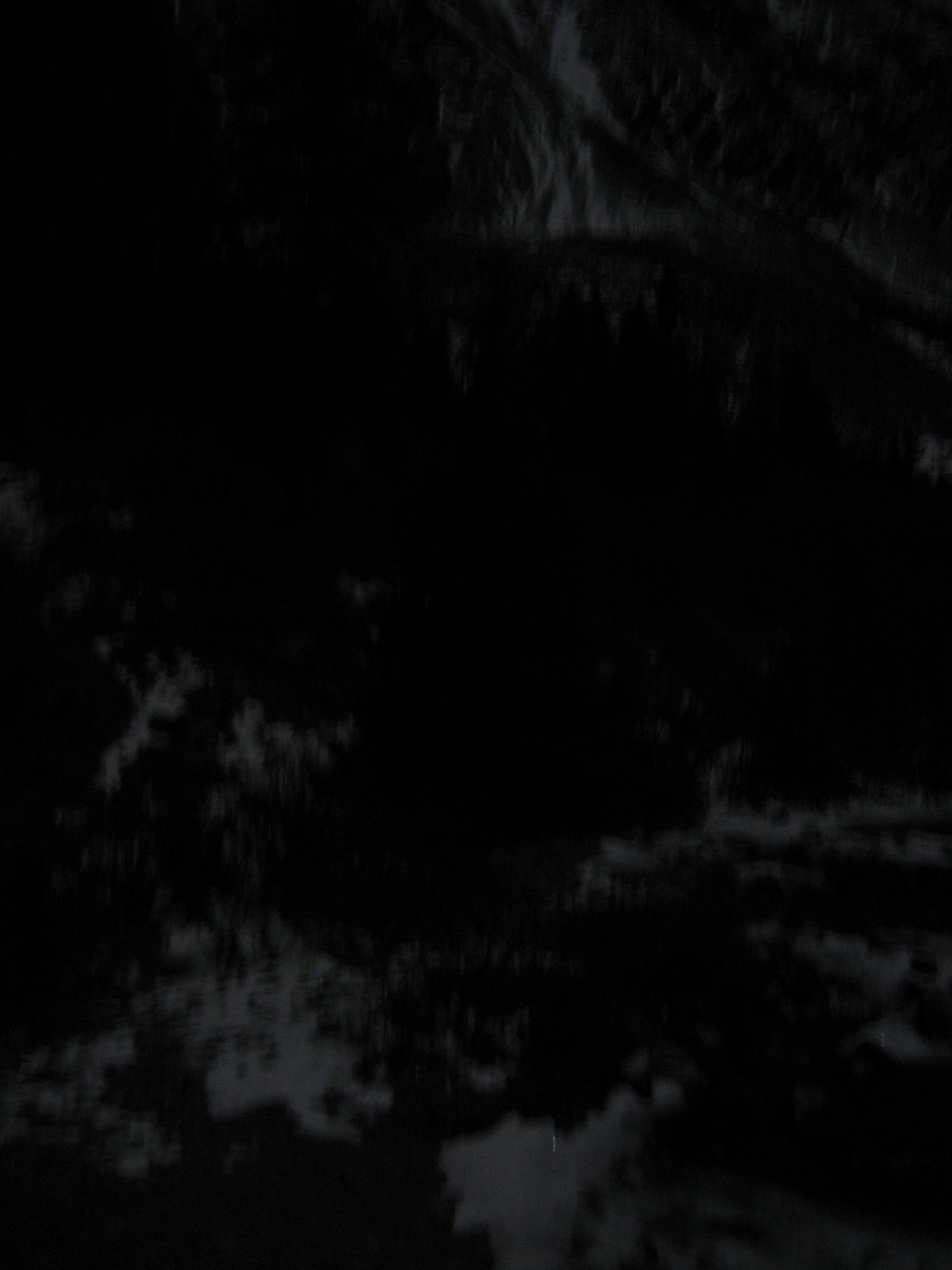A confusing and blurred image, predominantly pitch-black and highly distorted, offers a mysterious and ambiguous scene. No flash was used, rendering the center completely obscured in darkness. The only discernible element is in the top right corner, where what appears to be a rock or stone wall can be seen. This hints at a potential setting—perhaps within a cave system or at the entrance to a dark alcove beneath a mountain. The central black mass might contain water, possibly evident by faint reflections that suggest the presence of tree tops beneath the stone wall. This intriguing composition leaves much to the imagination, inviting viewers to ponder its true nature.